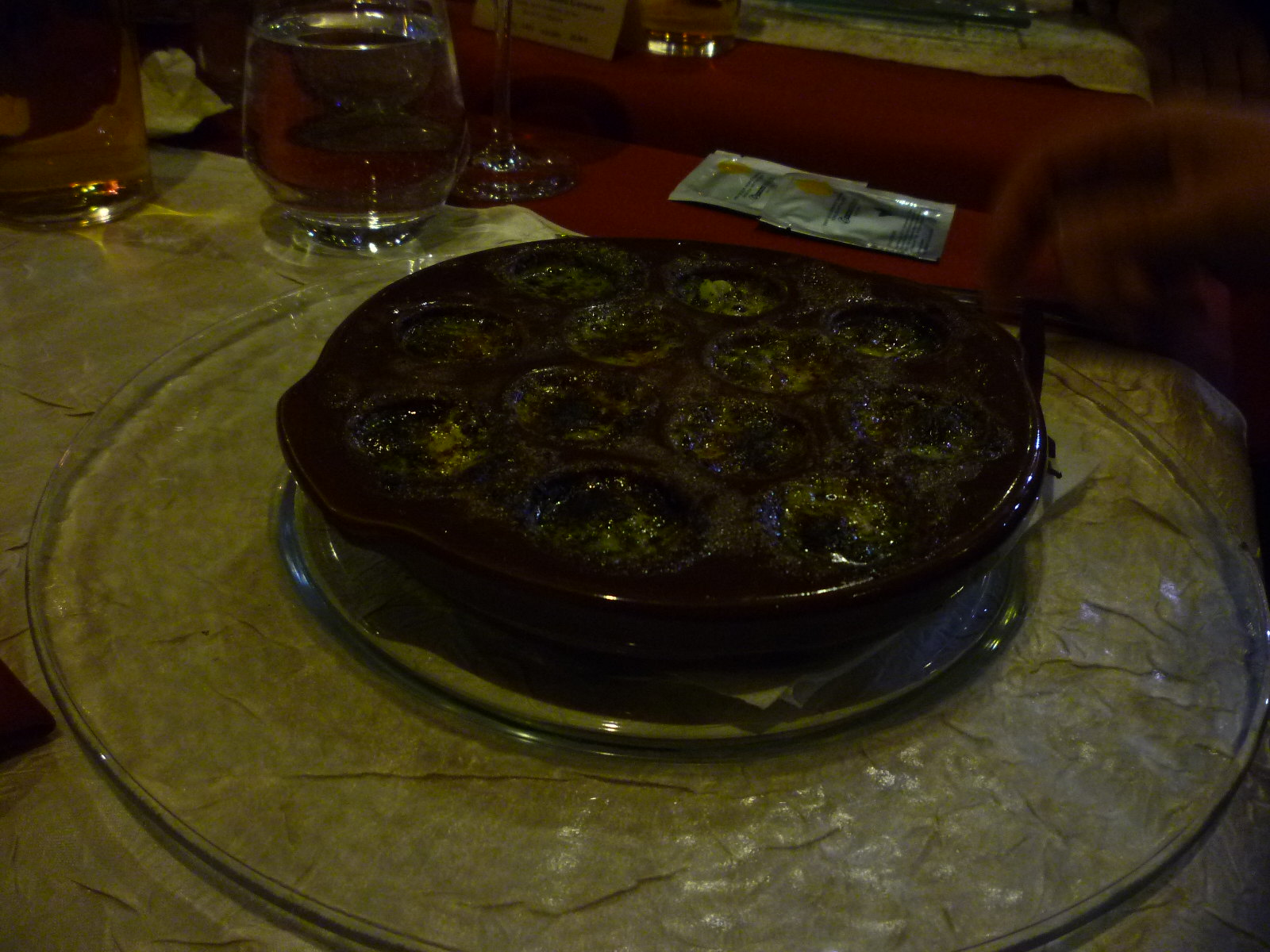In this photograph taken in a dimly lit restaurant, a dark brown ceramic dish with multiple circular compartments, reminiscent of an escargot plate, is prominently featured. Each compartment of the dish appears filled with a dark, indistinguishable substance that could potentially be covered with cheese and herbs. The ceramic dish is placed on a larger glass turntable or plate that sits atop a white or beige tablecloth. In the background, there are two silver packets, likely containing hand wipes, a glass of water, a tall glass stemware, and a blurred hand resting near the tablecloth, adding a human element to the scene. The overall low lighting contributes to the difficulty in discerning the finer details of the food, enhancing the mysterious and cozy ambiance of the setting.